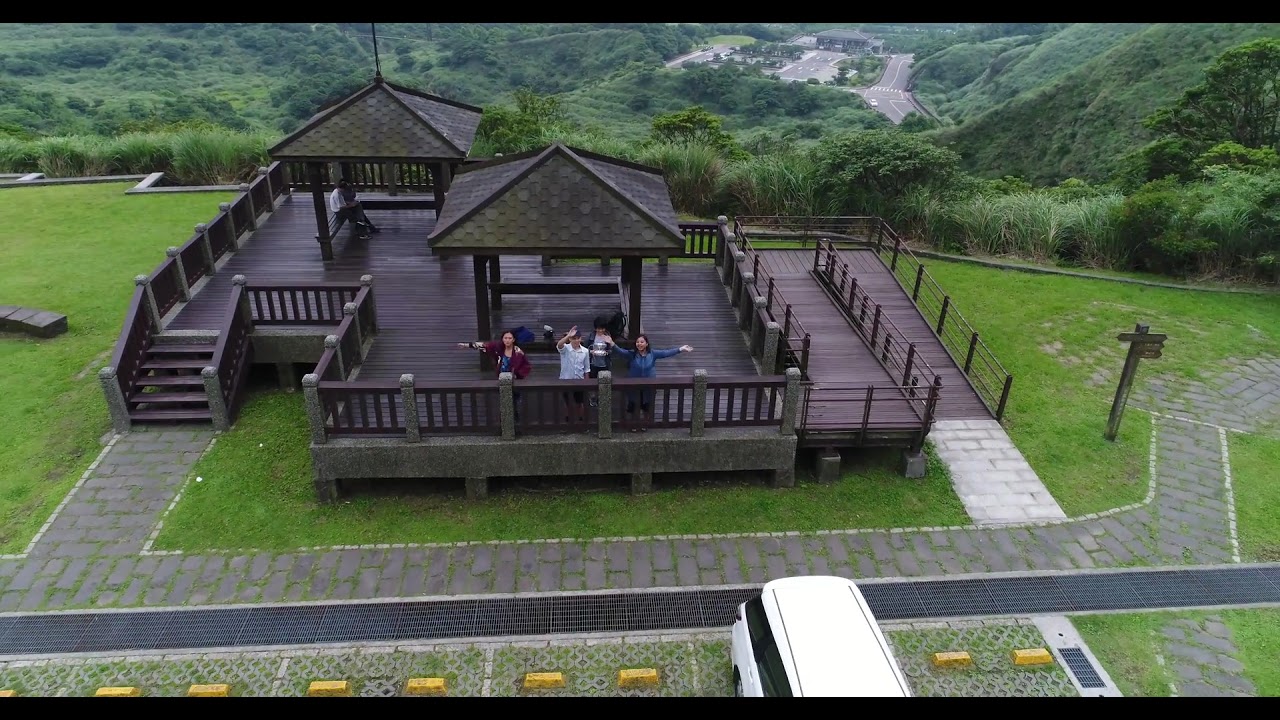In a drone-captured image on a gloomy day, the scene showcases a large, wooden, and stone-crafted pavilion within a park, featuring two roofed canopy areas resembling gazebos. The pavilion includes both a left-side stairway and a right-side wheelchair ramp, bordered with a fence, which descends toward a sprawling area of grass and vegetation, hinting at a valley below. The foreground is marked by a stone pathway parallel to a parking lot, where a white van is parked. In front of the pavilion, four people are posed facing the camera: a girl in a red or maroon jacket, a man in a white shirt with his hand raised in a wave, another girl in a blue jacket with her arms extended joyously, and a boy slightly behind them, engrossed in a silver object in his hand. In the distance, clusters of trees frame the background, completing this serene, slightly rainy outdoor setting.